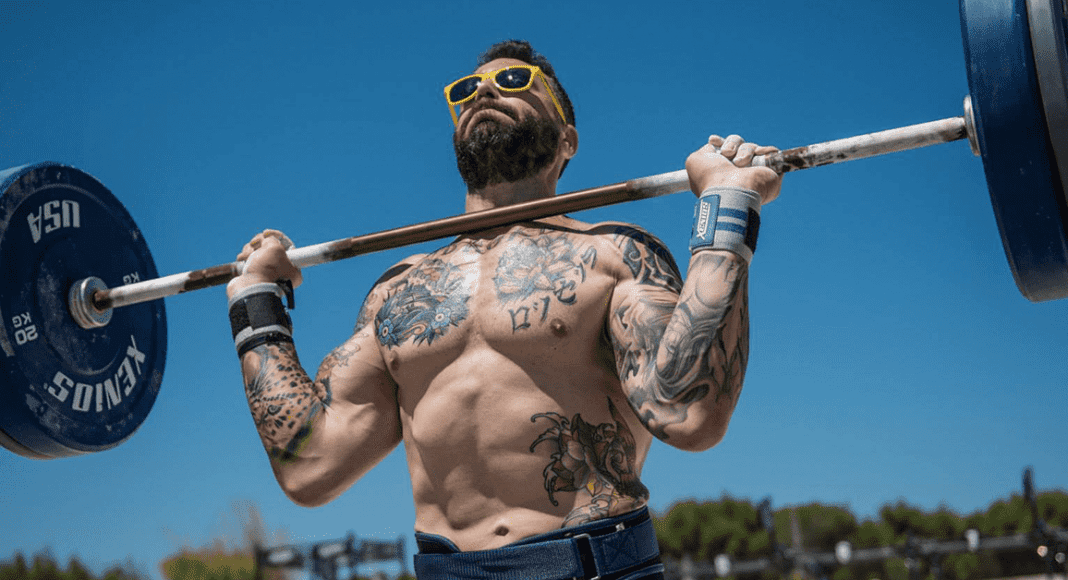The image captures a very muscular man with a beard, mustache, and thinning brown hair, standing outdoors under a clear blue sky. He is wearing yellow-framed sunglasses and a weightlifting belt around his waist. The man is adorned with numerous tattoos on his chest, the left side of his torso, and both arms. He's gripping a barbell with a brown and white handle, and blue weights on each end inscribed with "XENIOS USA" and "20 KG" in white ink. His hands, which are supported by wrist straps, hold the barbell at chest level, poised to lift it further. The bright daylight and a backdrop of blurred green vegetation enhance the scene, emphasizing his defined muscles and focused stance.